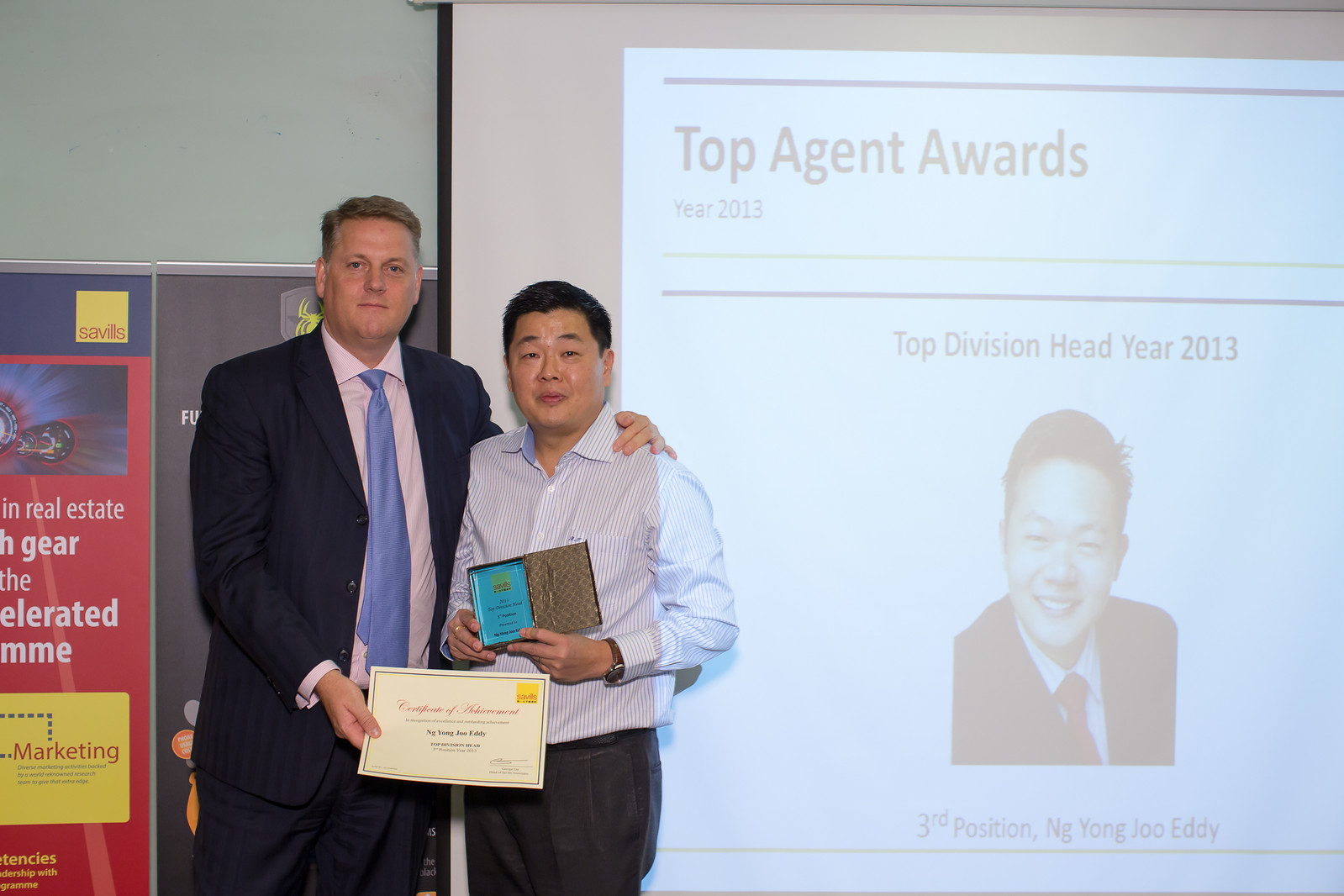The photograph features two men in an indoor setting, likely at an awards presentation. On the left is a Caucasian man with light brown hair, dressed in a blue business suit, light pink button-up shirt, and a light blue tie. He is holding a certificate of achievement in his right hand, with his left arm wrapped around the other man. The certificate bears the name Enjong Juedi. The man to the right, Enjong Juedi, has black hair and is wearing black pants, a blue and white checkered long-sleeve shirt with a collar, and a black wristwatch on his left wrist. He is holding a flat, gold-colored award with a blue rectangle in his hands. Behind them is a projection screen displaying the text "Top Agent Awards, Top Division Head, Year 2013," along with a picture of Enjong Juedi, noting his achievement in the third position.